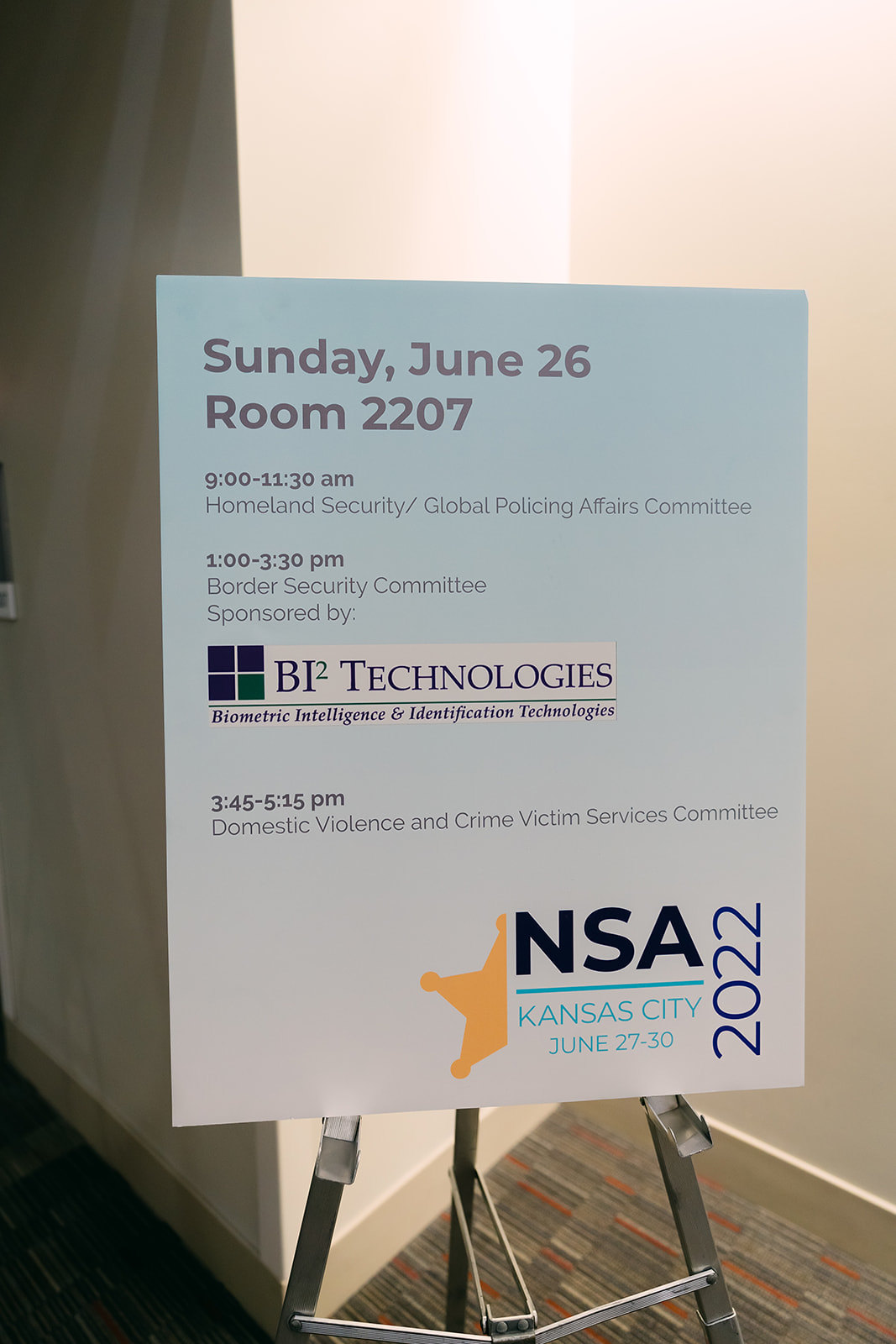The image is a detailed photograph of a gradient blue signboard promoting an event schedule, mounted on a three-legged metal stand that can be folded up. The gradient blue background of the signboard transitions from light blue at the top to white at the bottom.

At the top of the signboard, in large black text, it reads: "Sunday, June 26th, Room 2207." Below this, in smaller black text, the schedule of events is laid out:

- 9:00 to 11:30 AM: Homeland Security / Global Policing Affairs Committee
- 1:00 to 3:30 PM: Border Security Committee sponsored by BI Squared Technologies, Biometric Intelligence, and Identification Technologies
- 3:45 to 5:15 PM: Domestic Violence and Crime Victim Services Committee

In the bottom right corner of the signboard, "NSA" is written in dark font next to half of a sheriff's badge. Below the "NSA," running vertically, it says: "Kansas City, June 27th - 30, 2022."

The photograph seems to have been taken inside a building, likely at a conference, with the signboard placed against whitewashed walls in the corner of a room, although there isn't much else visible in the photograph.